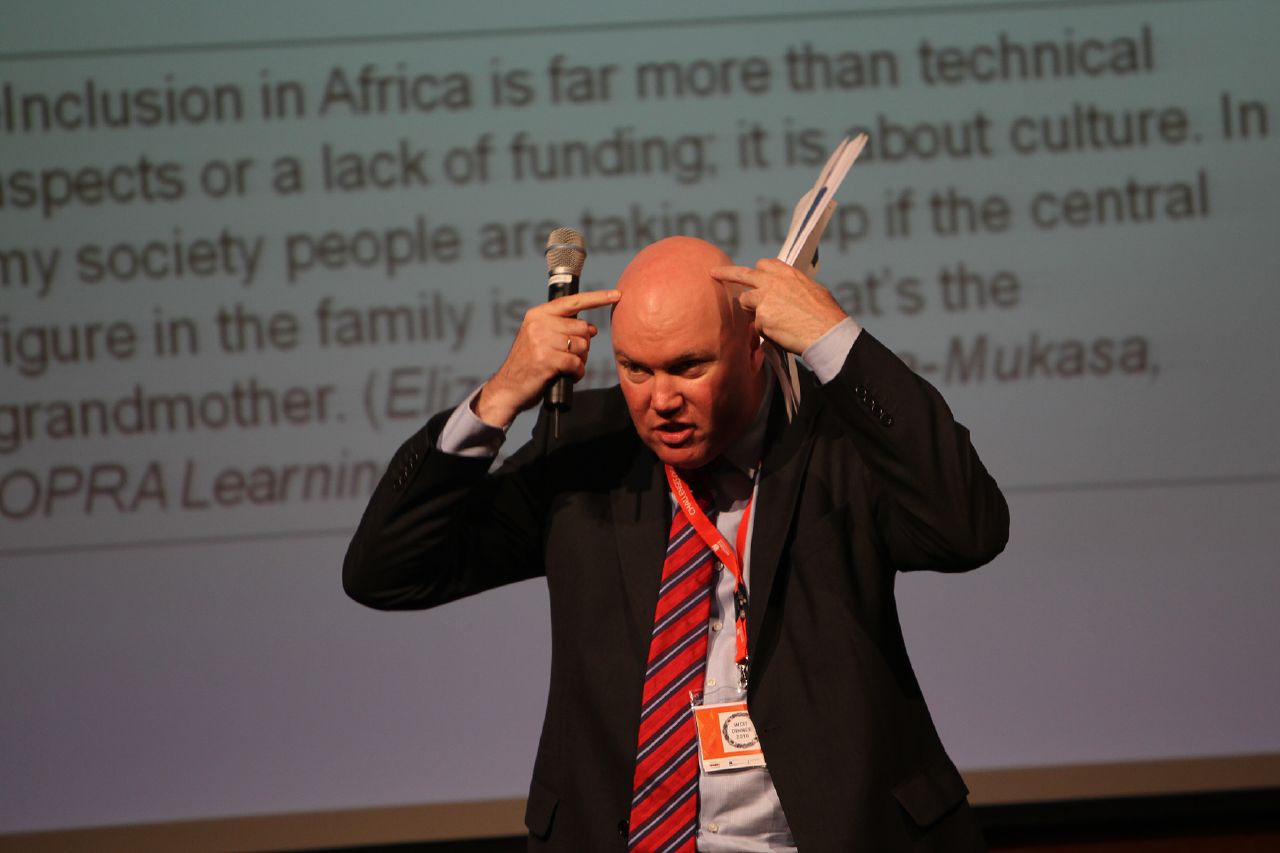The photograph captures a bald man intensely speaking at an event, seemingly emphasizing a critical point. He is dressed in a dark suit jacket over a light-colored shirt, paired with a red and blue striped tie. A red lanyard with a name badge or participant badge hangs around his neck. The man, who has a wedding ring on his left hand, holds a microphone in that hand while clutching a packet of papers in his right. Both hands are raised to his head with his index finger from the right hand and the middle finger from the left hand touching his forehead, indicating a moment of deep contemplation or emphasis. His serious expression is directed towards the audience. In the background, a projector screen displays a slide with a white background and bold black text in a black box, partially visible but conveying a message about the cultural aspects of inclusion in Africa. The text reads: "Inclusion in Africa is far more than technical aspects or lack of funding. It's about the culture. In my society, people are taking it up as the central figure in the family is …" however, some parts of the text are obscured.